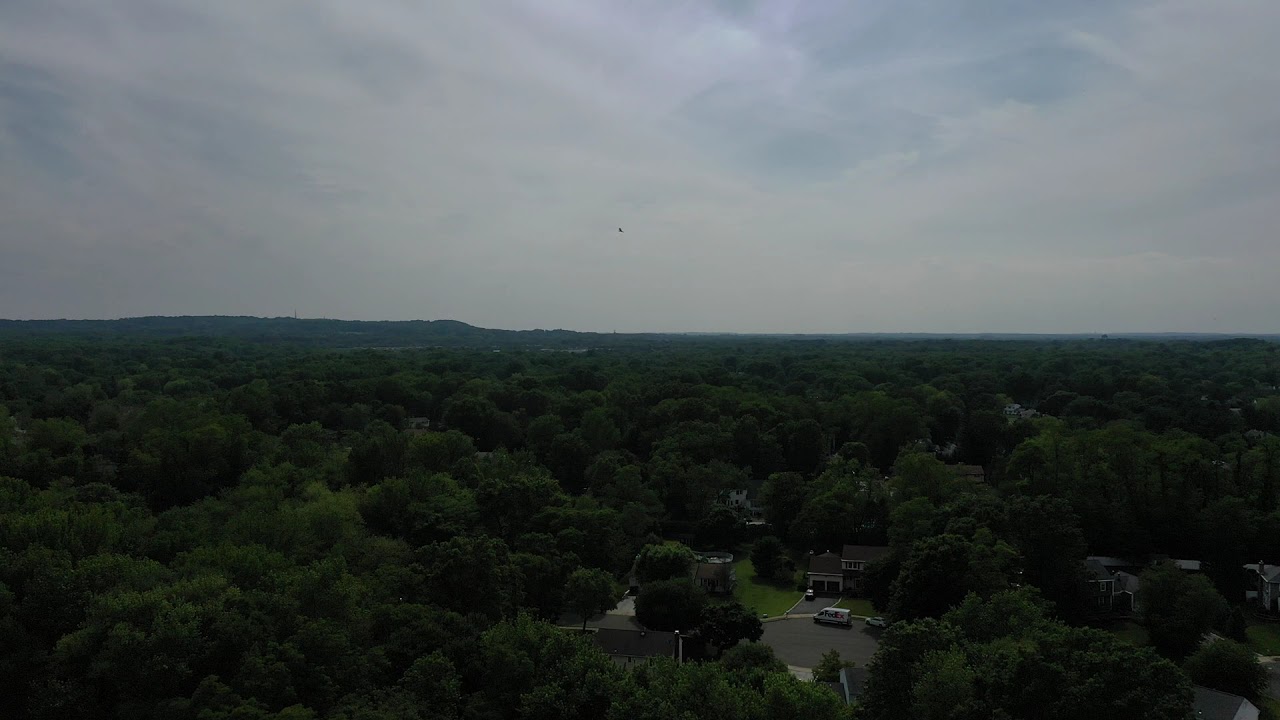The image captures an overcast aerial view of a densely treed area with dark green foliage under a gray, cloudy sky. The horizon features rolling hills and stretches halfway across the image, contributing to the overall somber lighting. In the bottom center, a small clearing reveals a house with a driveway, where a car is parked. A FedEx van is positioned on the adjacent street, pointing towards the left. The presence of additional homes and structures is hinted at through the dense trees, indicating a suburban or urban setting. Despite the heavy tree coverage, some streetlights and small poles are visible, adding subtle illumination to the relatively dark scene.